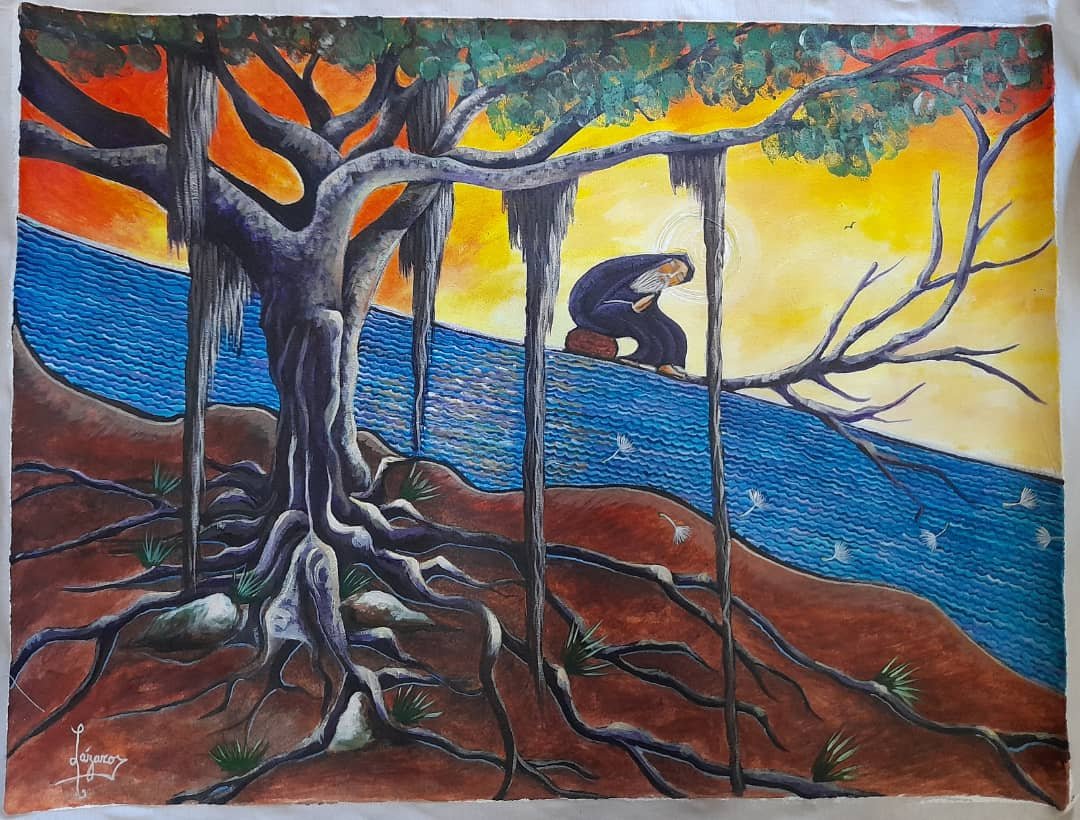This surreal and modern painting by Lazaro Chabalos depicts a serene landscape in vivid color. On the left, a gnarled gray tree with moss draping down its branches stands prominently above its tangled roots sprawling across the deep brown earth. Sparse green leaves crown the tree, adding a touch of life to its aged trunk. The scene shifts to a tranquil waterside setting in the background, indicated by rippling blue lines. At the water's edge, an elderly man with a long white beard, dressed in a blue robe, is seated on a brown object that appears to be a log. He leans forward, his feet resting on a branch that stretches out into the water. Behind him, the sky is a brilliant canvas of glowing yellow and deep orange hues, suggesting a mesmerizing sunset. The composition is marked by its stylized approach, blending natural and fantastical elements to create a serene tableau inspired by the Psalms. A bright halo-like ring behind the man’s head further accentuates the ethereal quality of the scene.